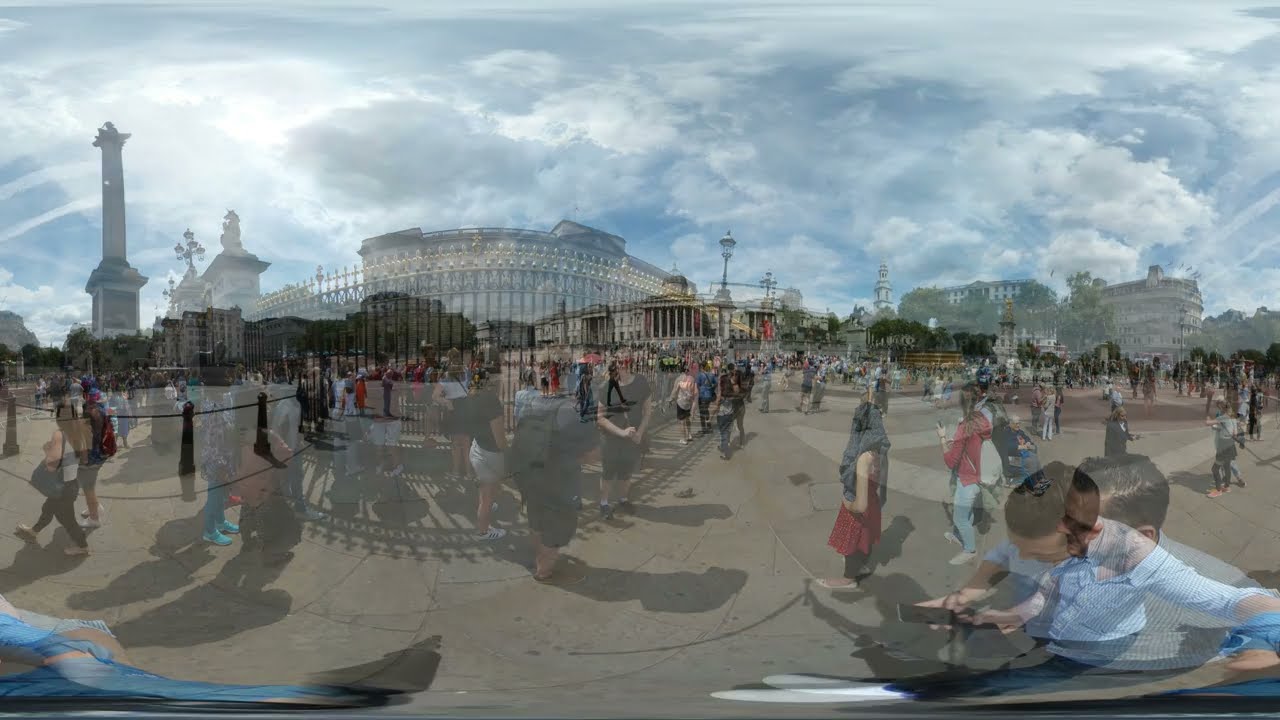The image depicts a bustling city square, teeming with pedestrians traversing a vast, open paved courtyard. The ground is adorned with an intricate arrangement of square stone pathways in varying shades of gray. Dominating the middle of the image is a prominent building with grand Greek architecture, featuring imposing pillars and heavy structural designs, evoking a sense of officialdom or historical significance. On the left side, a monumental decorative pillar stands tall, with intricate engravings, providing a focal point for several onlookers. Nearby, people are gathered around a fountain with a golden base, adding a touch of elegance to the urban setting. Amidst the crowd, in the foreground, a man is absorbed in his phone, epitomizing the busy yet casual vibe of the place. The composition, captured in a panoramic shot, reveals more old structures and lush trees in the background, framed by a sky filled with clouds, lending a serene contrast to the lively scene below.